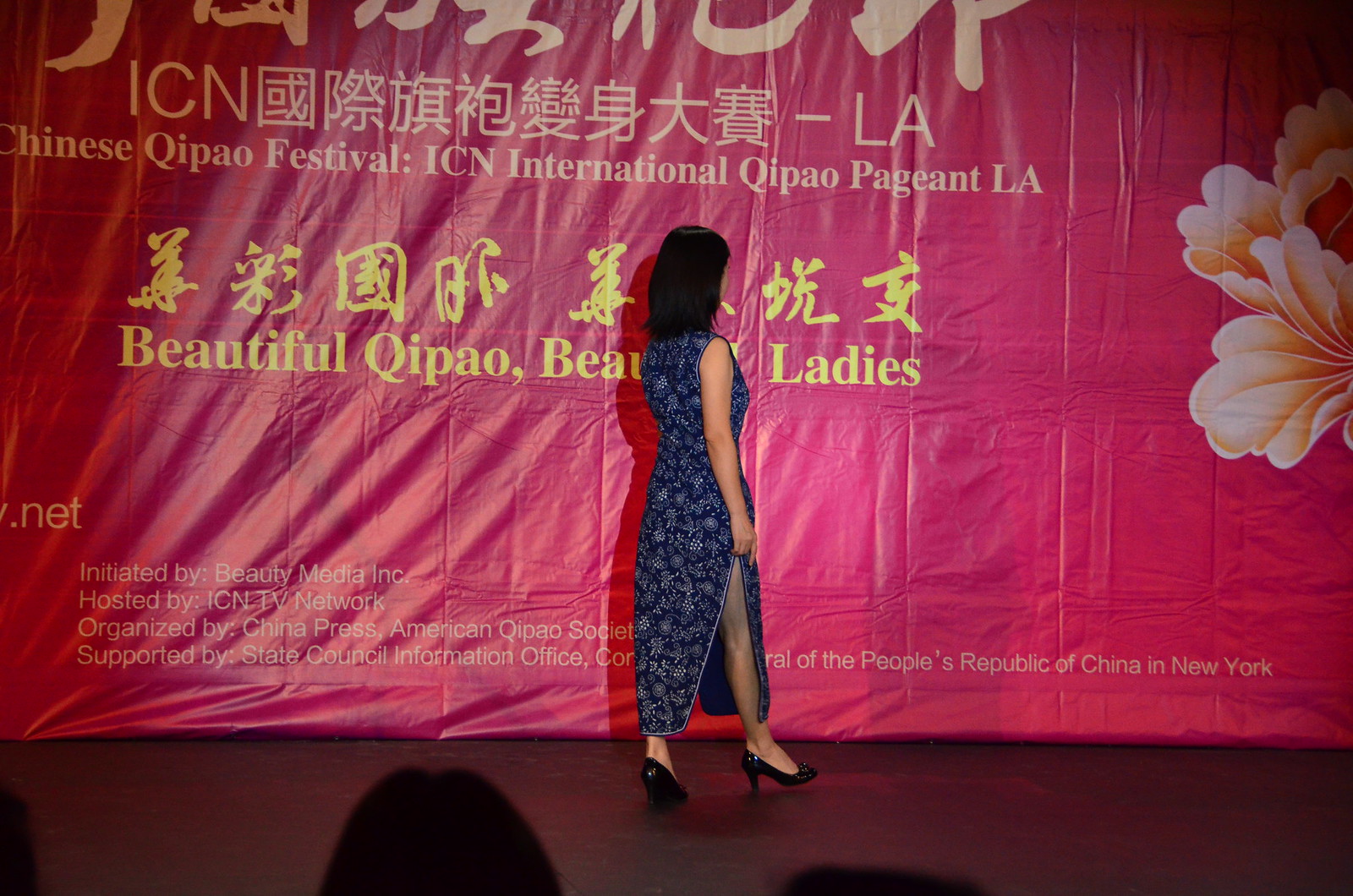The image captures an Asian woman in the midst of a beauty pageant, walking gracefully across a stage, her side profile illuminated by a spotlight. She dons a floor-length, sleeveless dark blue dress adorned with a white floral pattern, which features a high slit revealing her leg. She wears black high heels and her shoulder-length, straight black hair swings gently as she moves. The background is dominated by a large pinkish-red banner adorned with Chinese characters and English text. The banner announces the "Chinese Qipao Festival ICN International Qipao Pageant LA," and includes phrases like "Beautiful Qipao, Beautiful Ladies." It also features a large white flower on the right side. Additional text at the bottom left of the banner credits the event's sponsors: “Initiated by Beauty Media Inc., hosted by ICN TV Network, organized by China Press American Qipao Society, supported by State Council Information Office of the People’s Republic of China in New York.” In the foreground, the tops of two audience members' heads are seen in silhouette, hinting at the presence of spectators engrossed in the event.